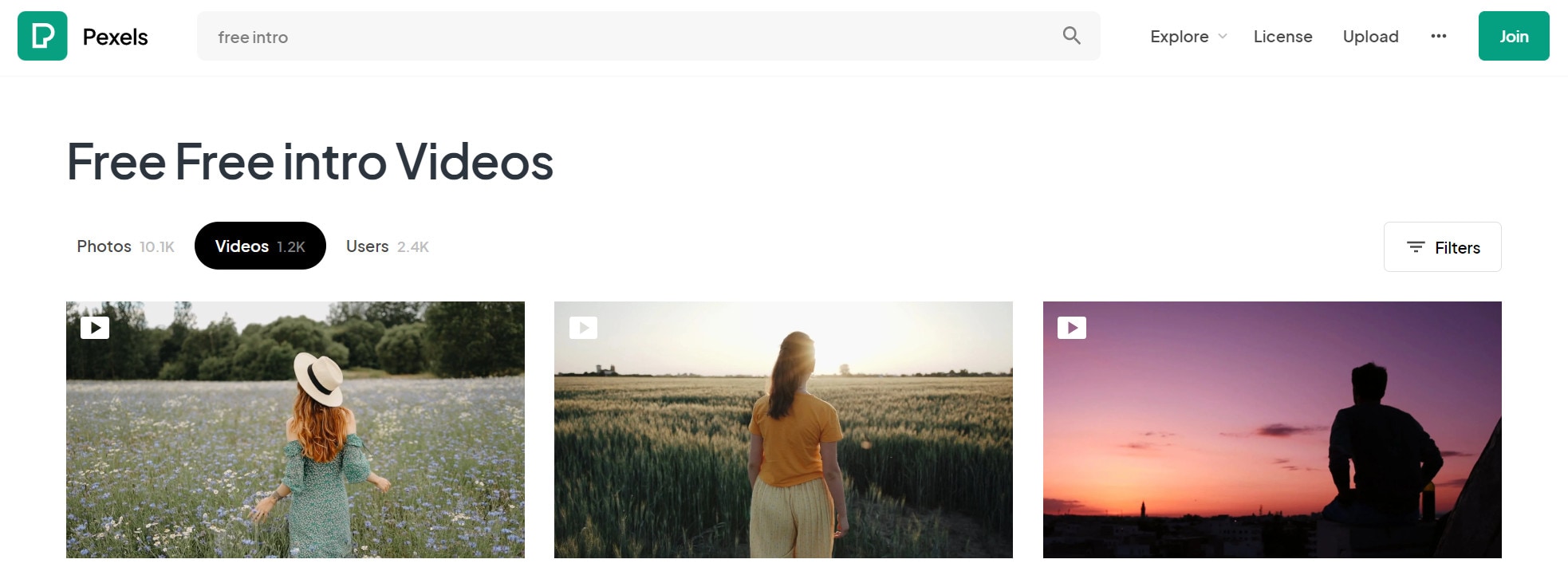The image features a clean white background with several elements scattered across the layout. On the left side, there is a green section with white lettering showing the letter 'P', adjacent to the word "pixels" in black. A grey box containing the text "free intro" is flanked by a magnifying glass icon on the right. Further to the right, a series of options are listed in black font: "explore," "arrow down," "license," "upload," "three dots," and "join," with the latter situated within a green box.

Below this header section, the left side displays "free intro videos" in larger black font, while "photos 10-16" appears in much smaller black font underneath. To the right, a black circle containing "videos 1.2k" in white font is visible, next to another section showing "users 2.4k" in black font on a white background.

The main section includes three video thumbnails:
1. The first thumbnail on the left shows a landscape with green trees and tall grass. A red-haired woman wearing a white hat with a black rim and a green dress is visible. This thumbnail is marked by a black arrow on a white background in the top left corner.
2. The second thumbnail features a woman in an orange top and white checkered pants standing in a tall green field. She gazes out at a grey sky during either sunset or sunrise.
3. The third thumbnail on the right captures a person sitting and leaning forward, bathed in a vibrant gradient of purple on the right and yellow-orange hues on the left. The person is silhouetted against the background, looking at a sunset, with a hint of black at the bottom of the image.